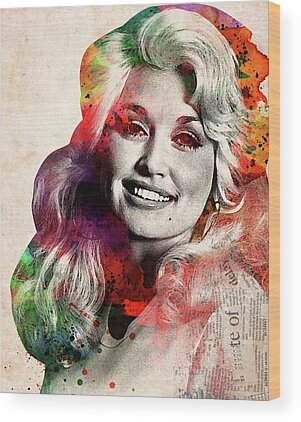This is a computer-generated portrait of a young Dolly Parton, showcasing her iconic long blonde hair, which is infused with vibrant colors like green, purple, yellow, orange, and red, giving it an abstract appeal. Her face appears predominantly in black and white, reminiscent of a newspaper photo, with a distinct mole near her mouth accentuating her bright, toothy smile. The portrait is set against a gradient background with shades of gray and peach, and features scattered text elements resembling newspaper print on the lower right corner. Dolly is depicted wearing a white shirt amidst colorful splatters, including vivid pink on the left side, adding to the dynamic, collage-like aesthetic of the artwork. The entire composition is presented on a canvas, lending it a 3D texture and depth.